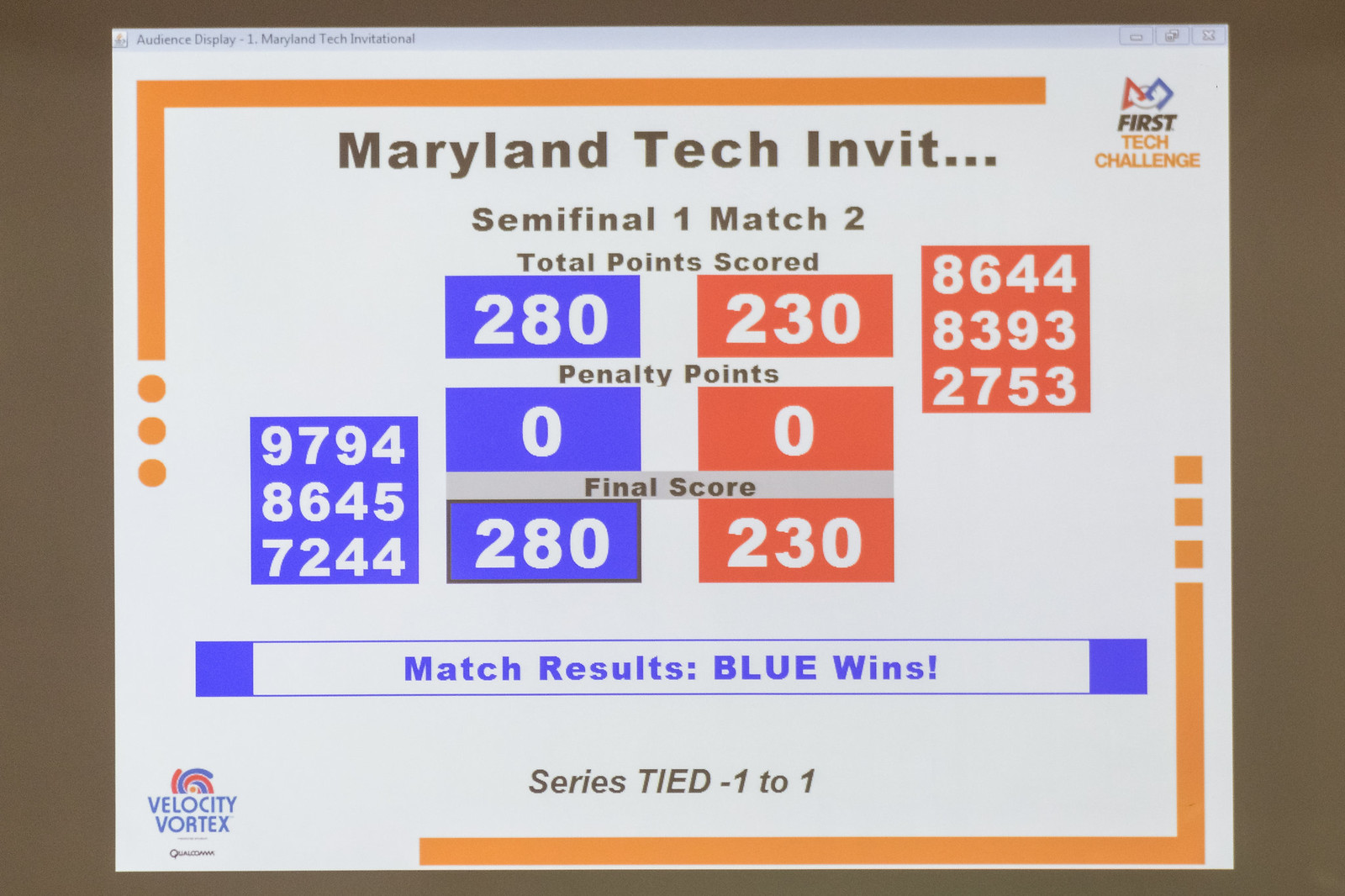This image presents a detailed screenshot of a computer display, most likely taken in a Windows 7 environment, reminiscent of audience presentation software. The screenshot centers on the Maryland Tech Invitational, specifically highlighting a First Tech Challenge semi-final match (Match 2 of Semi-Final 1). The title bar features an icon that resembles the Java logo, and the headline reads "Audience Display - 1 Maryland Tech Invitational". 

Against a clean white background, the main body shows the match's details: Blue team versus Red team, with the Blue team scoring 280 points against the Red team's 230 points. Both teams have zero penalty points, with the final score confirming the Blue team's win. Consequently, the series is tied at 1-1. 

Complementing the main display, there are colored boxes on either side containing team numbers. The left side (Blue team) lists the numbers 9794, 8645, and 7244. Meanwhile, the right side (Red team) features the numbers 8644, 8393, and 2753. Additionally, the display includes two logos: the First Tech Challenge logo in the top right corner and the Velocity Vortex logo in the bottom left corner. A blue banner across the bottom reinforces the result, inscribed with "Match Results: Blue Wins, Series Tied 1-1" in small black text. Orange lines accentuate the left-hand corner and the right-hand bottom corner, adding a visual cue to the presentation layout.